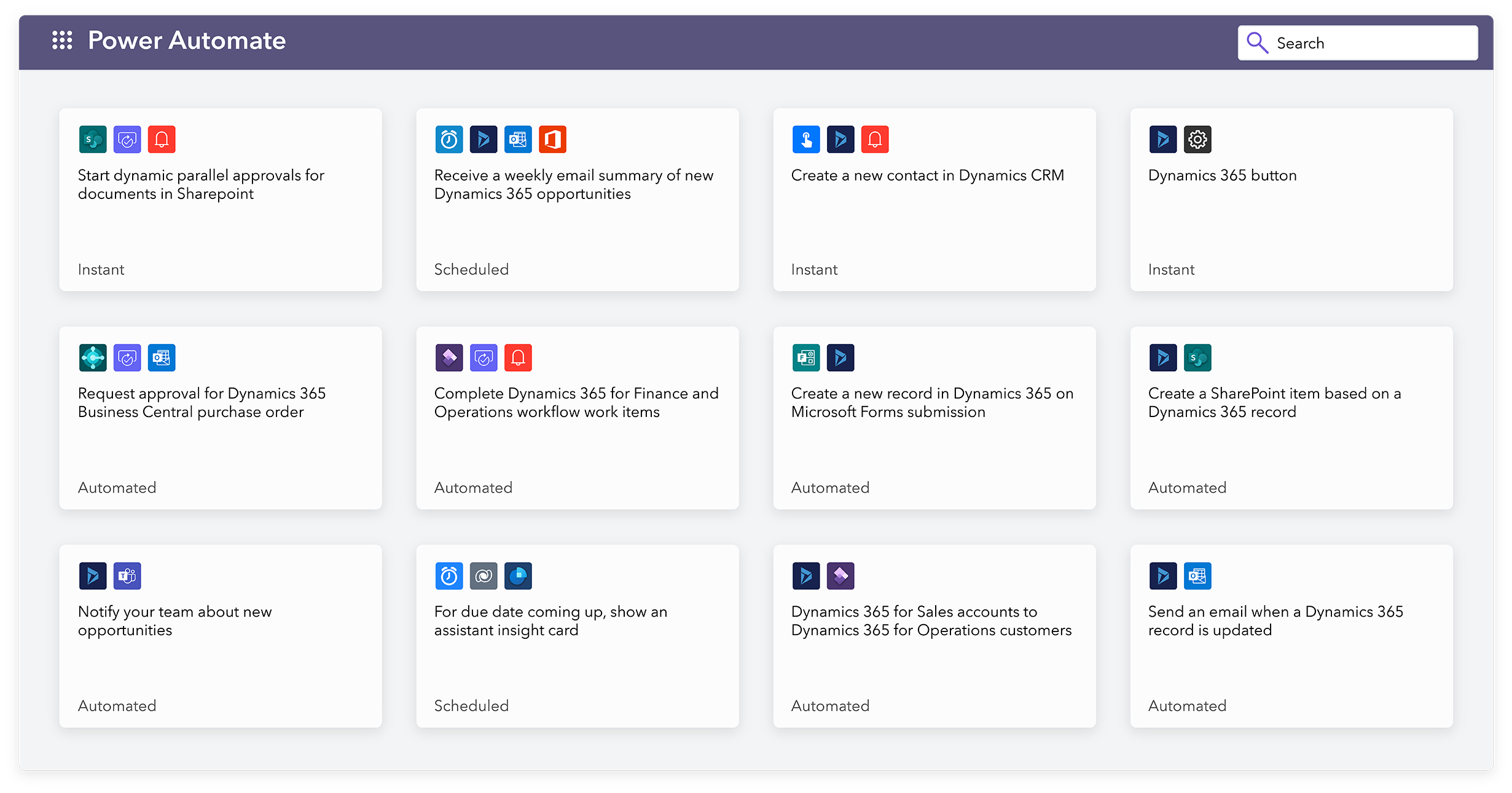The image showcases a screenshot of a website with "Power Automate" displayed prominently in the top left corner. A purple-colored bar spans the top of the webpage. On the far right of this bar is a white search box featuring a magnifying glass icon on the left side. Beneath this, the background shifts to white, populated by a grid of white cube-shaped tiles arranged in a 4x3 format, totaling 12 tiles. Each tile features an icon at the top, with text below providing additional information. At the bottom of each tile, the schedule status for various processes is listed. The first row shows statuses as "Instant", "Scheduled", "Instant", and "Instant". The second row displays "Automated" for all four tiles. The third row indicates "Automated", "Scheduled", and "Automated" for the last two tiles.